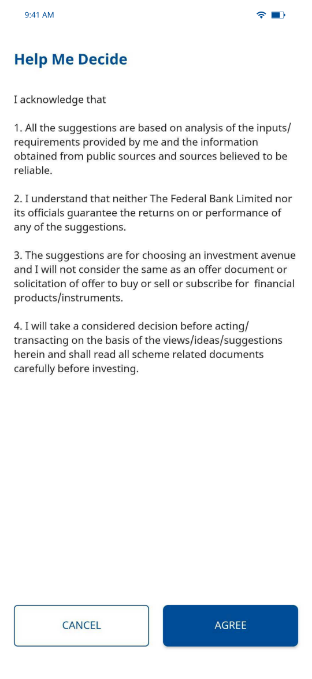The image is a screenshot taken from a mobile device at 9:41 AM, as indicated in the top left corner. The Wi-Fi signal icon, displaying full connectivity, is positioned in the top right corner. The main content of the screenshot centers on an interface, likely from a financial or investment-related app or website.

At the top of the interface, in bold blue text, it reads, "Help Me Design." Below this, a lengthy disclaimer is written in gray text, stating several conditions and acknowledgements the user must agree to before proceeding. The key points of the disclaimer include:

1. The suggestions provided are based on an analysis of the user's input requirements and information obtained from public and believed-to-be reliable sources.
2. The user understands that neither "the federal," "bank," "limited," nor its officials guarantee the returns or performance of any suggestions provided.
3. The suggestions are meant for choosing an investment avenue and should not be considered an offer document or a solicitation for buying, selling, or subscribing to financial products such as instruments.
4. The user agrees to make a considered decision rather than acting solely based on the suggestions, views, or ideas provided. Additionally, they must read all scheme-related documents before investing.

The disclaimer continues with additional points, but they are not fully visible in the screenshot.

Overall, the caption reflects the meticulous disclosure requirements typical in financial advisory applications, emphasizing the importance of informed decision-making and the limitations of liability on the part of the advisors.